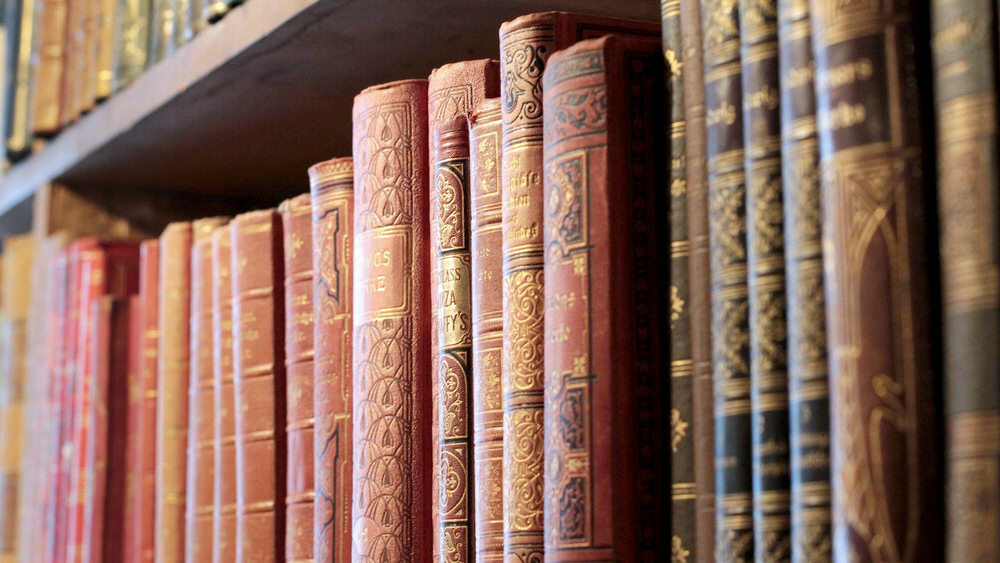In this close-up photograph of a bookshelf, the arrangement of books creates a stunning visual gradient, transitioning from pinkish-red on the left to brown on the right. The books on the left are smaller and become larger and clearer in focus toward the right. The aligned spines display intricate gold writing and filigree, with many featuring decorative patterns and scrollwork. The texture and appearance of the books suggest that they might be religious volumes, perhaps bibles, given the detailed designs and the resemblance to classic religious texts. The spines predominantly showcase dark red and brown hues, lending a rich, vintage ambiance. The brown shelf above, seen at an angle, adds to the stylized nature of the image, enhancing its visual appeal and depth.